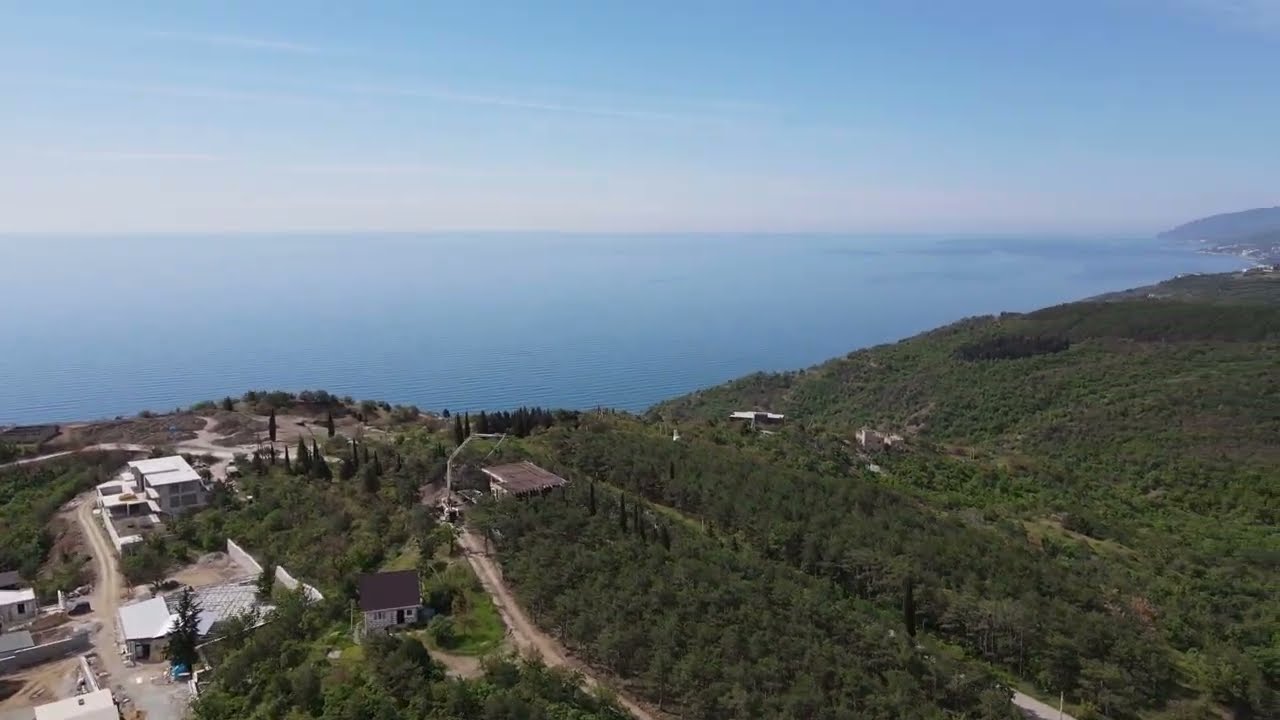The horizontally aligned rectangular photo captures a breathtaking aerial perspective of a diverse landscape blending natural and man-made elements. The upper portion of the image showcases a clear blue sky adorned with streaky, stradiated white clouds. Below the sky, a vast body of water, possibly an ocean or a large lake, stretches across the middle of the frame, exhibiting a grayish-blue tint with subtle ripples.

In the bottom half, the land is predominantly forested, featuring a thick canopy of trees. The terrain is hilly but flattens out towards the right side into grassy areas. Scattered across this lush vegetation are a few dirt roads and several buildings. On the left side, a white building, which might be a small factory or business, and a possible house with a brown roof, stand out. The right side includes a couple more white buildings, one of which could be a multi-story house or a small hotel. Despite the presence of these structures, there's an evident lack of human activity as no people or cars are visible, except for a single, vaguely discernible parked vehicle. The overall scene creates a harmonious balance between nature and development, viewed from a serene, elevated vantage point.